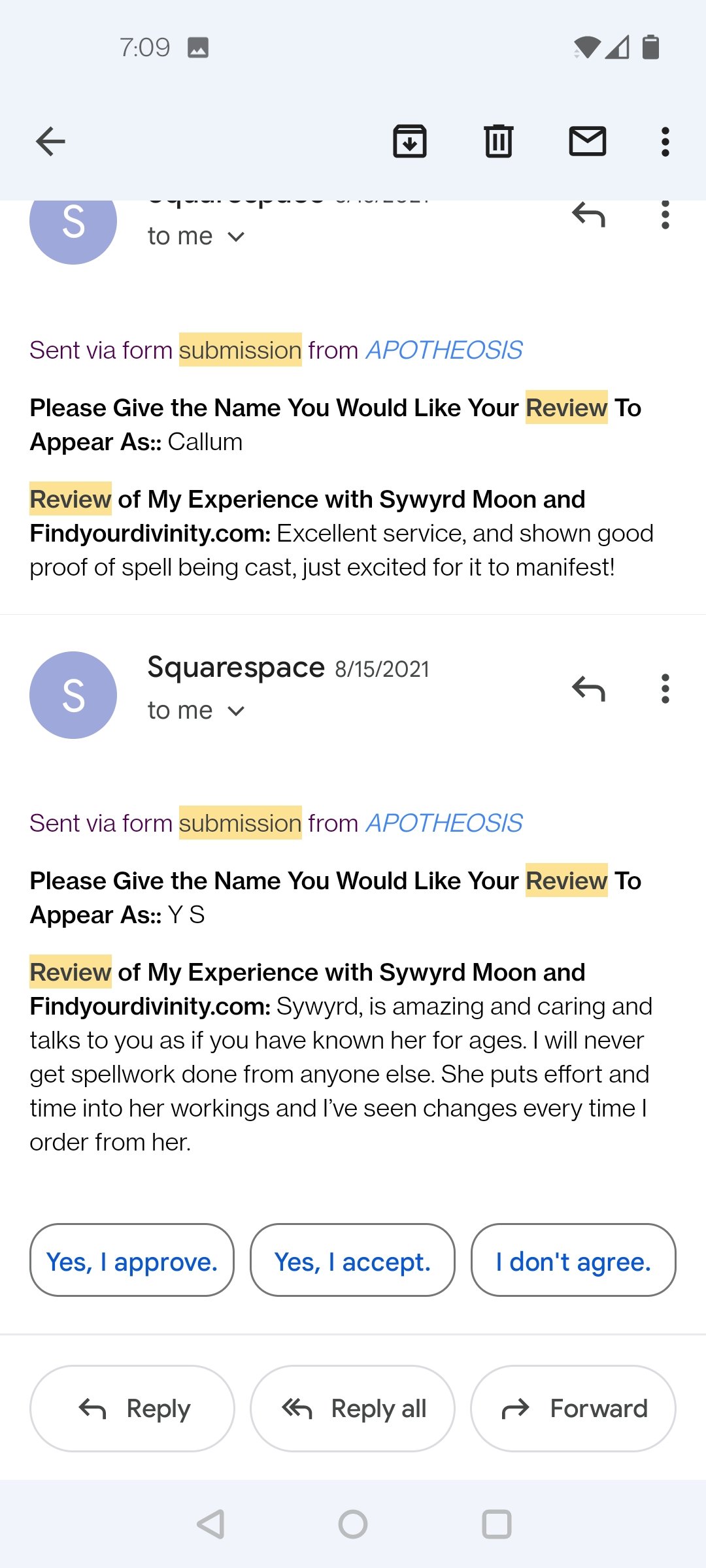The image displays a phone screen showing an email interface typical of Gmail. At the top, standard phone status icons are visible, including the time, Wi-Fi signal, and battery life indicators. Below, a left arrow, a download button (depicted as a file with a downward arrow), a trash icon, a mail icon, and a menu represented by three dots are present.

The main body of the email reads as follows:

---
**From:** Tim Mee (represented by an 'S' in a blue circle)   
**Subject:** Sent via form submission (highlighted in yellow)   
---
**Content:**  
Preview (highlighted in yellow)  
Review of my experience with Cyword Moon and findyourowndivinity.com

"Excellent service and showing good proof of spell being cast."

From SquarePace on August 15th to Tim Mee:  
"Sent from submission. Please give the name you would like your review to appear as: YS."  

The reviewer states:  
"Cyword is amazing and caring and talks to you as if you have known her for ages. I will never get spell work done from anybody else. She puts effort into her work, and I've always seen changes every time I order from her."

At the bottom of the email, there are options to respond, including 'Yes, I approve,' 'Yes, I accept,' or 'I don't agree.' Additionally, reply, reply all, and forward buttons are visible.